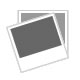The image features a striking artistic style with a predominantly black background highlighted with shades of grey. Central to the illustration is a meticulously depicted wine glass filled with a vibrant pink liquid and a maraschino cherry at the bottom. At the top of the glass, the text "Cocktail Recipe" is elegantly inscribed in white. Superimposed on the wine glass is the phrase "Pink Lady" displayed in a stylish white font, embellished with pink outlines. Below the glass, a dotted line stretches horizontally across the image, segmenting it. Under this line, the ingredients for the cocktail are listed in precise white text: one and a half ounces of gin, half an ounce of apple jack, half an ounce of freshly squeezed lemon juice, half an ounce of grenadine, one small egg white, and a maraschino cherry garnish. The harmonious combination of text and imagery creates an inviting and visually appealing recipe illustration.